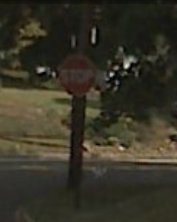In this blurry image, a stop sign stands prominently at the corner of a residential street, bordered by a concrete curb. On the right side of the frame, the branches of a tree partially obscure the view, while more branches appear on the left, possibly from a different tree. Directly behind the stop sign, the residential lot on the corner features a glimpse of a parked car. Across the street, a well-kept lawn leads up to a driveway where another vehicle is visible, suggesting the presence of a home just beyond the view of the camera. The street surface transitions seamlessly from asphalt to the concrete curbing, emphasizing the typical suburban setting.